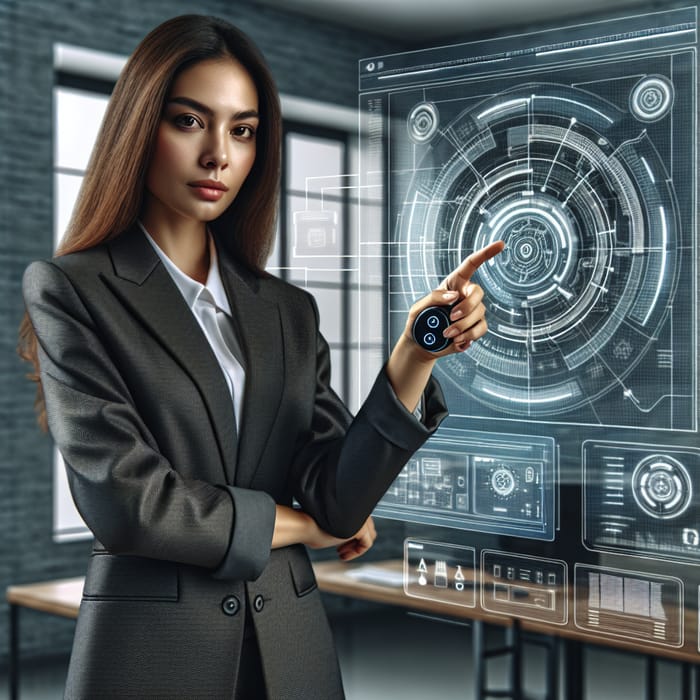The image showcases a digitally created, elegant young woman, possibly of Asian or Hispanic descent, with long, dark hair cascading past her shoulders. She stands confidently on the left side of the frame, looking directly at the viewer, wearing a sleek black suit jacket with partially rolled-up sleeves over a crisp white shirt. The setting is a technologically advanced room with a backdrop of grey brick walls and slightly blurred multi-pane windows that let in a soft light. 

She is pointing with her left hand at a sophisticated holographic projection floating in the air. This projection comprises a complex circular diagram, likely related to an advanced technical or scientific subject. The main circle contains smaller inner circles, with two additional circles in the top right corner and various transparent rectangles and other data beneath it. The futuristic display is replete with graphs and readouts, both analog and digital.

In her left hand, which she uses to gesture at the hologram, the woman holds a small black controller featuring two white buttons, one above the other. Below the projection, there is a modernistic brown wooden table supported by black metal legs, adding to the scene's sophisticated ambiance. The room's décor and the equipment suggest it is a cutting-edge lab or high-tech meeting room.